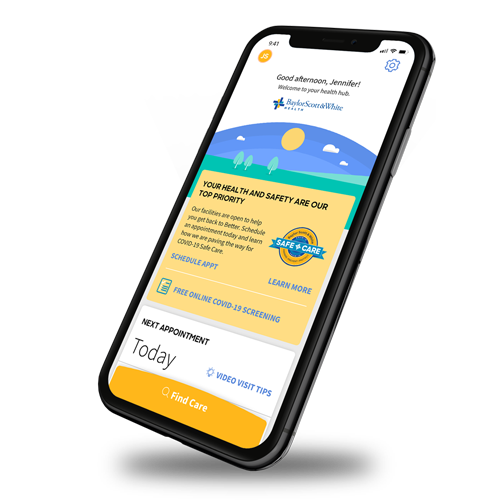In this image, a smartphone is positioned diagonally, displaying its screen prominently. The top of the screen reads, "Good Afternoon, Jennifer, Welcome to Your Health Hub," in a welcoming font. Below this text, there is a logo with illegible blue text. The background image on the screen depicts a serene field of green grass with three distinct trees standing tall. Above the field stretches a bright blue sky, almost dome-like, featuring a vibrant yellow sun and three fluffy white clouds.

Beneath this pastoral scene, a striking yellow box captures attention with the text, "Your health and safety are our top priority," written across the top. At the bottom of this yellow box, there are two buttons: "Schedule Appointment" situated on the left, and "Learn More" on the right, both inviting the user to take further action.